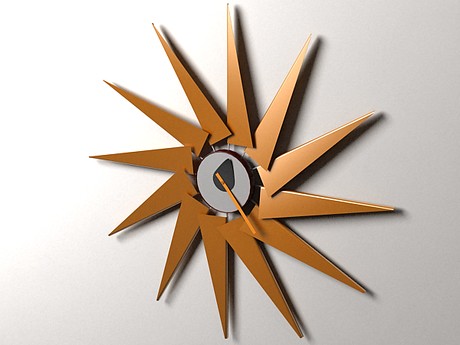This photograph features an abstract clock mounted on a wall, set against a background that transitions from white on the left to a medium gray on the right. The clock face is designed like a sunburst, with 12 golden triangular shapes radiating outward, closely resembling sails or sunrays, and slightly overlapping each other. These triangles help indicate the hours by pointing outward, with no numerical markers present.

The clock has two distinct hands: a long, slender brown minute hand and a short, black teardrop-shaped hour hand, resembling a guitar pick. The center of the clock features a small gray circle where both hands pivot. The clock's minimalist design is accentuated by a light source illuminating the left side, casting a subtle shadow on the right. To read the time, one must rely on the position of the hands and the triangular hour indicators, understanding the clock mechanics much like a traditional timepiece.